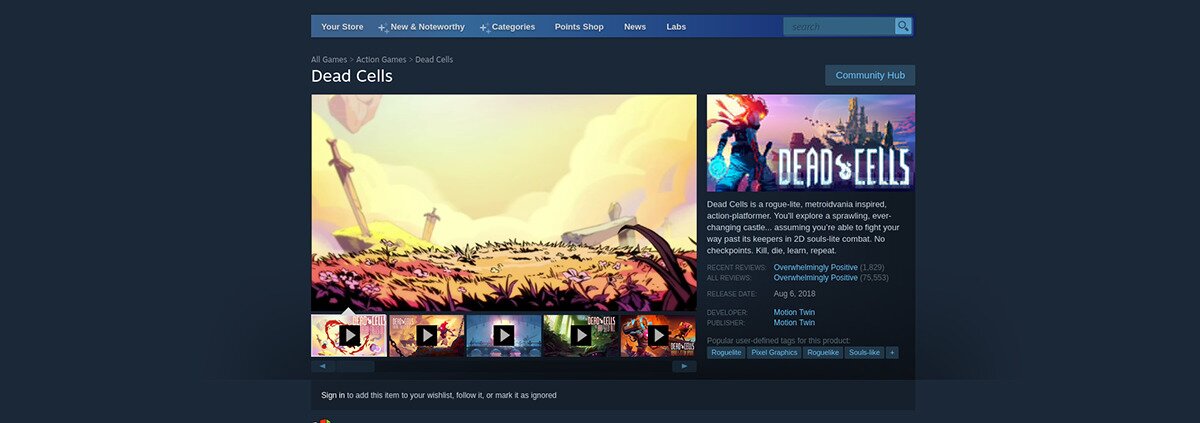The background of the image features a dark blue color with a blue search bar at the top. Below the search bar, in white text, is the title "Dead Cells." The sky depicted in the image is a vibrant yellow with scattered clouds. Emerging from a tall yellow rock are two long swords plunging down into it. The ground is a tan color interspersed with small black plants. There is also a red-hued area that contains a large axe lying on its side, appearing as if it is made of concrete.

To the right, in a distant secondary scene within the same image, a white castle is visible on the horizon. In the foreground of this scene, a strong, shadowy character is depicted carrying a weapon. Behind this character is a bright red backdrop resembling a meteor streaking across the sky. The character stands atop an area shaped like a blue heart. Flanking this scene, the words "DEAD CELLS" are prominently displayed in all capitalized white letters, with a plus sign inside a circle situated between the words "DEAD" and "CELLS."